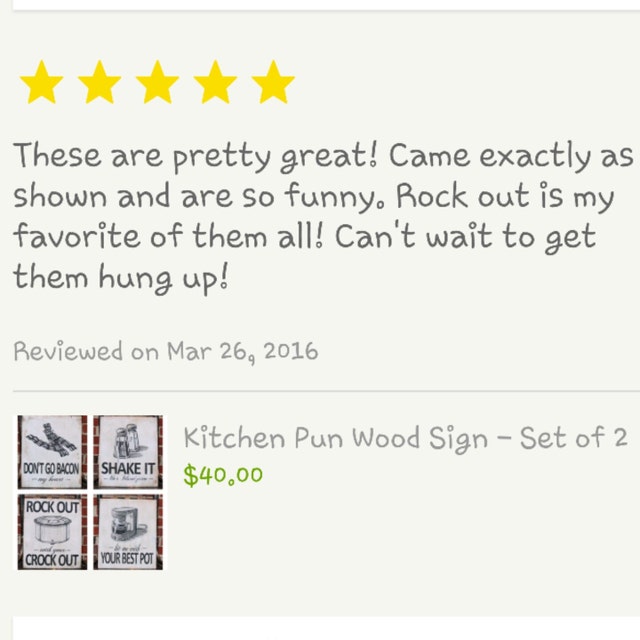This detailed descriptive caption accompanies a screenshot of a product review for a set of kitchen pun wood signs. At the top of the screenshot, five stars are highlighted, indicating a perfect rating. Below the stars, the reviewer praises the product, stating, "These are pretty great. Came exactly as shown and are so funny. 'Rock out' is my favorite of them all. Can't wait to get them hung up." The review is dated March 26, 2016.

The product in question is identified as "Kitchen Pun Wood Sign, Set of Two," priced at $40. To the left of the review text, there are four photographs of different signs, each featuring a black and white illustration accompanied by a humorous phrase. 

- The first sign depicts three slices of bacon with the caption, "Don't go bacon my heart."
- The second sign shows an image of a salt shaker and a pepper shaker with the phrase, "Shake it." The additional text underneath is too small to read.
- The third sign has an illustration of a crockpot with the phrase, "Rock out with your crock out."
- The final sign portrays a coffee maker with the words, "Hit me with your best pot."

The image contains no people, animals, plants, flowers, or trees.